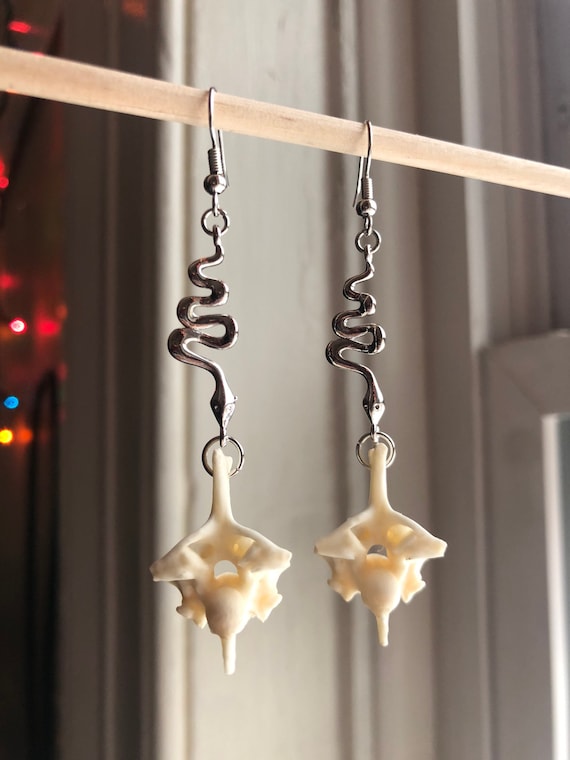The photograph captures a horizontally positioned, light tan wooden rod suspended indoors against a white wall background. Hanging from this rod are two ornaments that closely resemble earrings. Each ornament features a metal hook attached to a curvy, swiveled metal body reminiscent of a snake. At the bottom of these swiveled bodies, there's an ivory-colored, shark tooth-shaped object. The background of the image includes a portion of a window and is decorated with colorful Christmas lights in shades of red, blue, yellow, and orange.